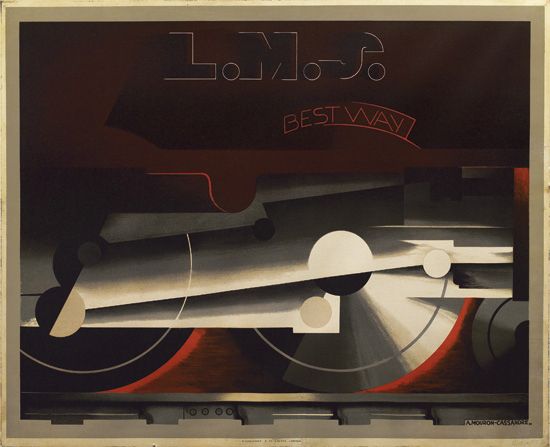This is a detailed and artistic poster featuring the abstract rendition of a locomotive train's wheels. Framed in a light beige border with a dark green backdrop, the image prominently displays the text "L.M.S." at the top in very dark red lettering, followed by "Best Way" in vivid red beneath it. The style evokes Art Deco influences, combining dark, rich colors like deep reds, browns, grays, and tans, interspersed with black and white elements. The composition appears to capture the train in motion, moving from left to right along a dark gray track, giving a dynamic feel to the poster. The two wheels, central to the image, are portrayed in contrasting colors – the left wheel in black with a red outline and the right wheel in a shiny silver with the same red edging. The wheels' bright stainless steel-like appearance adds a striking focal point to the artwork. Overall, it is a hand-drawn illustration with an abstract yet detailed aesthetic, celebrating the locomotive with a nostalgic and artistic flair.